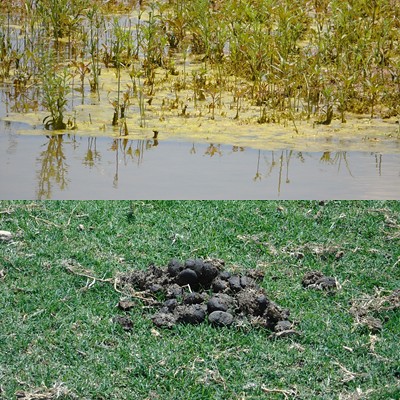This full-color photograph, taken outdoors on a sunny day, vividly captures a segment of nature split into two distinct sections. The lower part of the image showcases a grassy field, where the vibrant green grass is interspersed with patches of dead grass. Prominently in the center lies a substantial pile of dark, nearly black, animal dung composed of large balls. Ascending from this earthy foreground, the upper section of the photograph transitions to a serene body of water, resembling a swamp. The water's surface is adorned with pond scum and dotted with numerous green plants that rise above the waterline, their reflections shimmering on the surface. The photograph, marked by clear daylight, emphasizes the juxtaposition of grassy terrain and the tranquil, plant-rich water body, capturing the calm and complexity of a natural habitat.